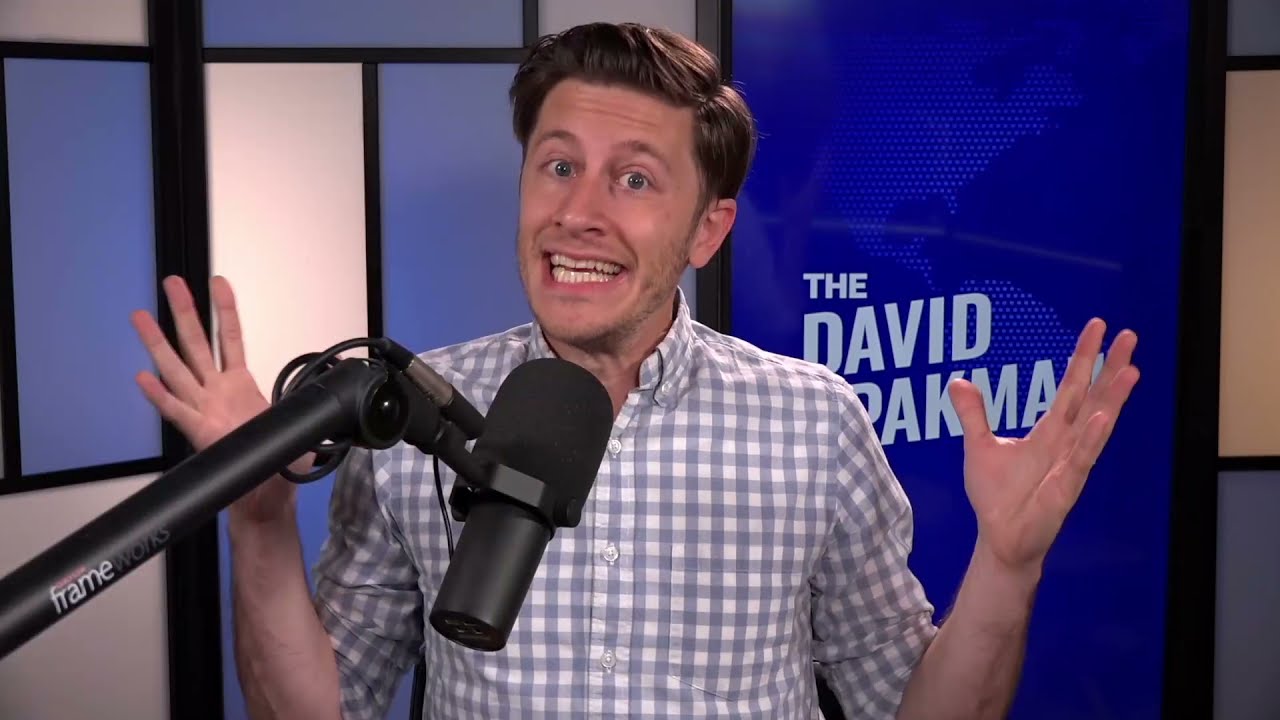The image captures David Pakman, likely during a recording session for his podcast or radio show. He's seated in front of a large black microphone on a stand angled towards his mouth. David's hands are raised to shoulder height, palms forward, and spread slightly away from his body. His facial expression is dynamic, with wide, emphatic eyes, crinkled forehead, and partially exposed, slightly yellow-tinted teeth. His eyebrows are raised, enhancing his expressive manner, and he appears to be speaking energetically. David's hair is neatly parted from left to right and styled with gel at the front. He is wearing a long-sleeved, white and gray checkered button-up shirt with the sleeves rolled up to his elbows. Behind him, a blue background features a globe motif and the name "The David Pakman Show" in white letters. The image is bright, clear, and high quality, suggesting a professional studio setting.